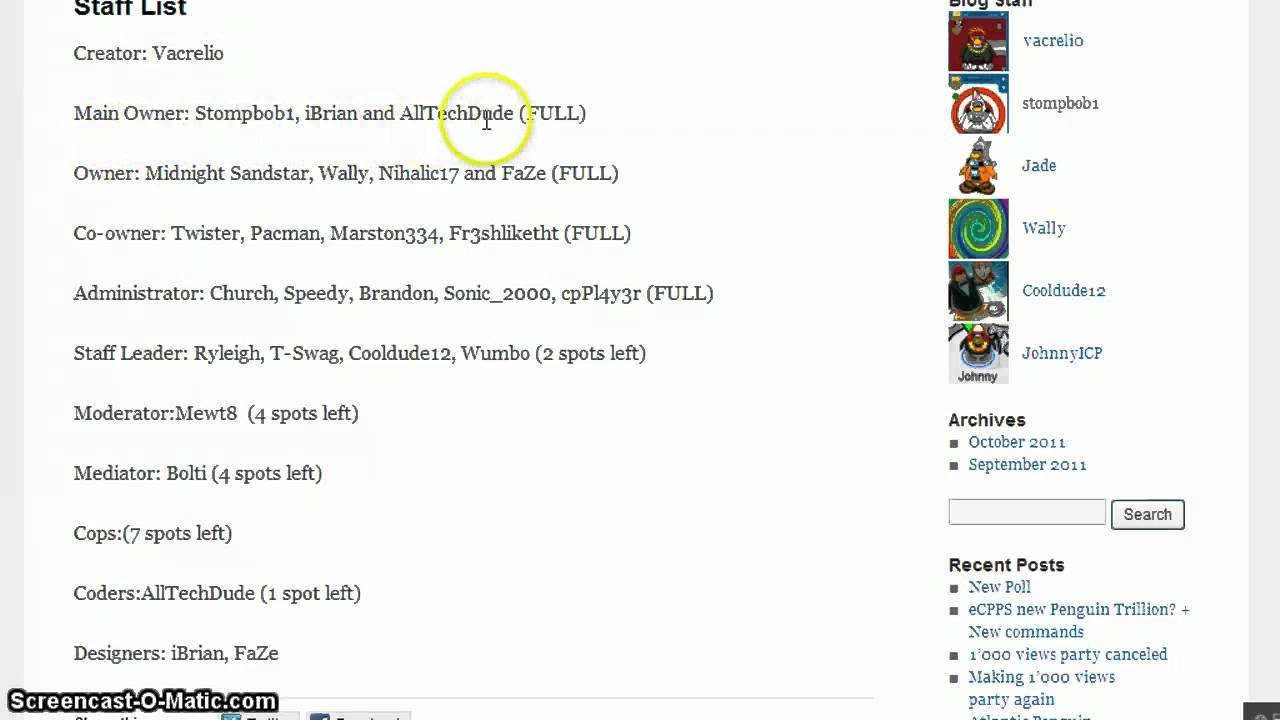A white-background web page screenshot in black font, bordered by gray vertical bars on both the right and left sides, akin to a forum website. At the top, the heading "Staff List" is in bold black font. Below this, a list of staff members is presented, categorized and itemized as follows:

- **Creator**: Varsiello, Main Owner: StompBob1, I, Brian, and All Tech Dude (Full) [circled in yellow]
  
- **Owner**: Midnight, Sandstar, Wally, Nahalik17, and FaZe (Full)
  
- **Co-Owner**: Twister, Pac-Man, Marston334, FreshLikeThat (Full)
  
- **Administrator**: Church, Speedy, Brandon, Sonic_2000, CP, Player3R (Full)
  
- **Staff Leader**: Riley, T-Swag, CoolDude12, Wumbo (Two spots left)
  
- **Moderator**: Mew, T8 (Four spots left)
  
- **Mediator**: Bolte